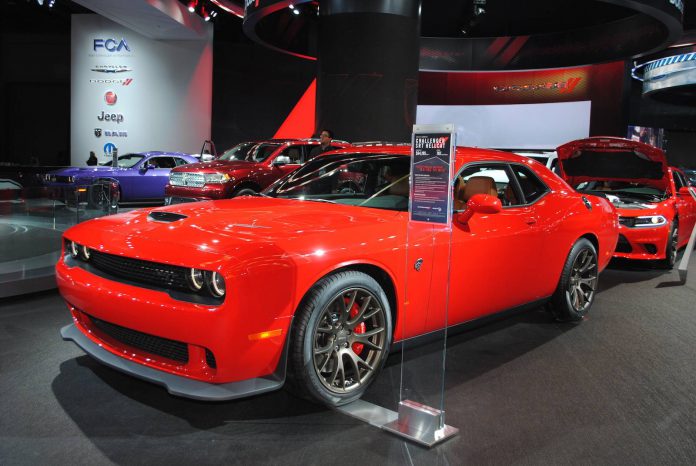The photo depicts a vivid red sports car showcased prominently in what appears to be a showroom or car exhibition hall, likely designed for showcasing automobiles. The car features silver wire wheels and distinctive black trim with gray accents, suggesting a blend of classic and modern design elements. This vehicle, possibly a Corvette or a similar American muscle car, is positioned near a sign with indiscernible text next to the driver's side door. The backdrop includes other vehicles, one of which is a red car with its hood open, and another that resembles an SUV. The interior of the showroom is adorned with flags and banners, and the walls prominently display logos such as FCA, Jeep, Chrysler, Dodge, and Fiat, among others, enhancing the ambiance of a formal car display or sales event. The overall setting is reminiscent of a convention hall or a sophisticated sales floor aimed at car enthusiasts and professionals.